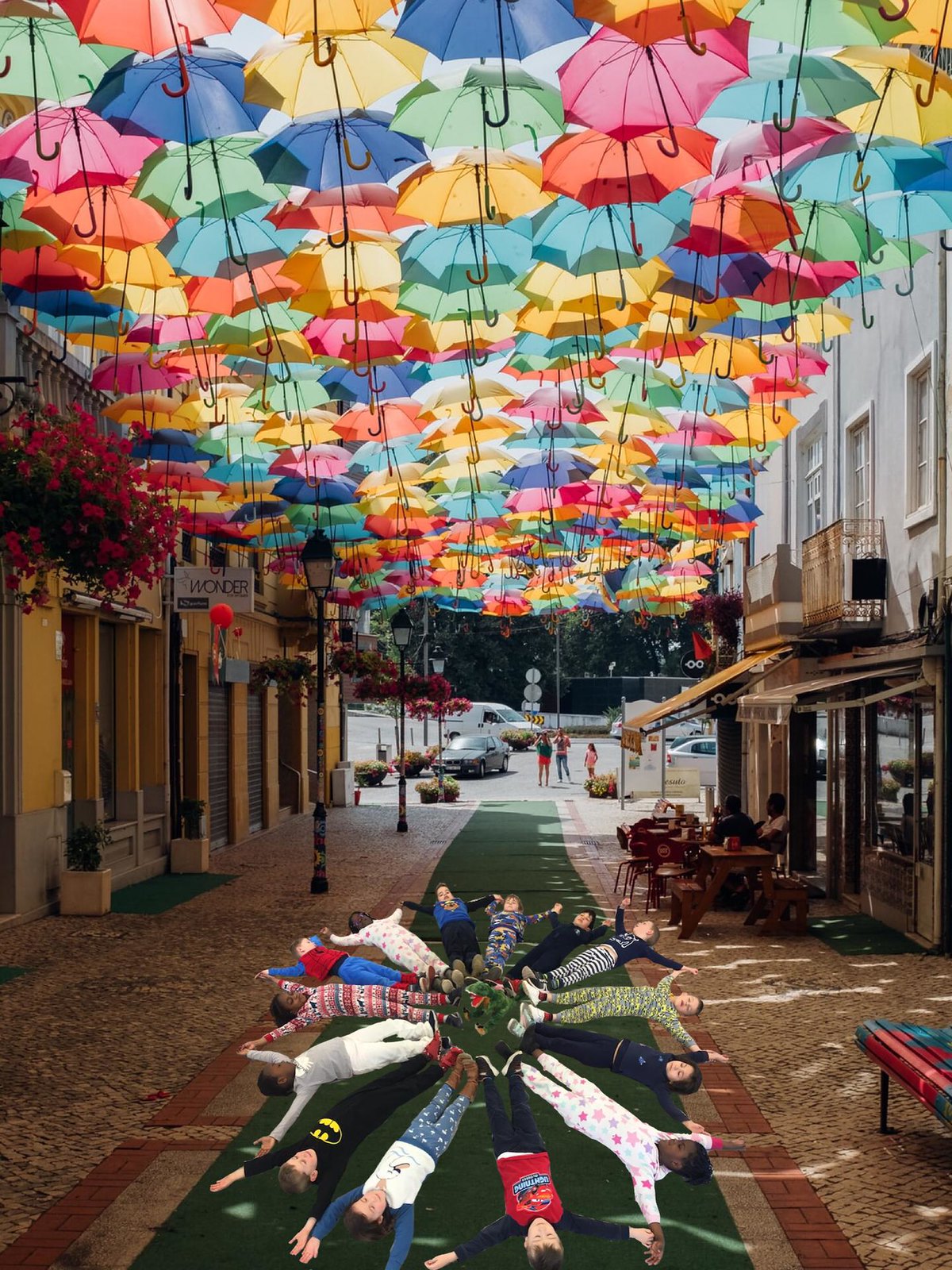This color photograph captures a whimsical and vibrant outdoor street scene. In the center of the image, about a dozen children are lying in a circle on a long emerald-green carpet that runs the length of the cobblestone-paved street. The children, dressed in a mix of colorful pajamas, with some in themed outfits like Batman and Spiderman, have their feet touching in the center and their arms stretched outwards, creating a star-like or floral pattern. The street is flanked by buildings, with a yellow one on the left and a grayish one on the right, housing businesses and some alfresco dining spots. Dominating the upper part of the image is a spectacular canopy of overlapping umbrellas in an array of colors—red, blue, green, orange, pink, and more—that extends across the entire width of the street, providing shade and a festive atmosphere. These umbrellas are semi-transparent and lit from behind by the sunlight. In the background, you can glimpse a few people standing, cars parked in a parking lot, and additional trees, adding depth to the scene.